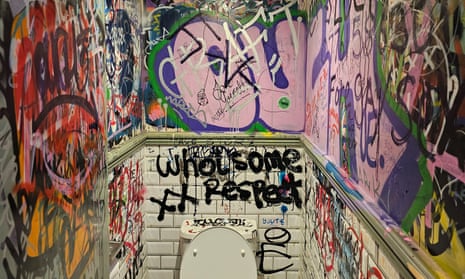The image depicts the interior of a public toilet stall, seen from the vantage point of someone who has just opened the door. The upper half of a white, rectangular toilet is partially visible, with the lid propped up against a cistern. The stall is replete with vivid and chaotic graffiti. 

The walls of the stall are divided visually; the top section, adorned with a wooden band running along three sides, is entirely saturated with a mélange of colors—pinks, blues, greens, and squiggles. The lower half features less dense graffiti on white ceramic tiles, which can still be glimpsed in patches on the left, right, and back walls. 

In the center of the back wall, directly above the toilet cistern, "Wholesome Respect" is prominently spray-painted in black, accented by two Xs. The left wall showcases a mix of reds, yellows, and blacks, with something resembling a man's head vaguely discernible in the mess. On the right side, amongst the pink and purple colors, one might make out "Cush" and "Large" amidst the chaotic scrawl. The door on the left edge of the image is also enveloped in vibrant graffiti, completing the tumultuous aesthetic of this public toilet stall.